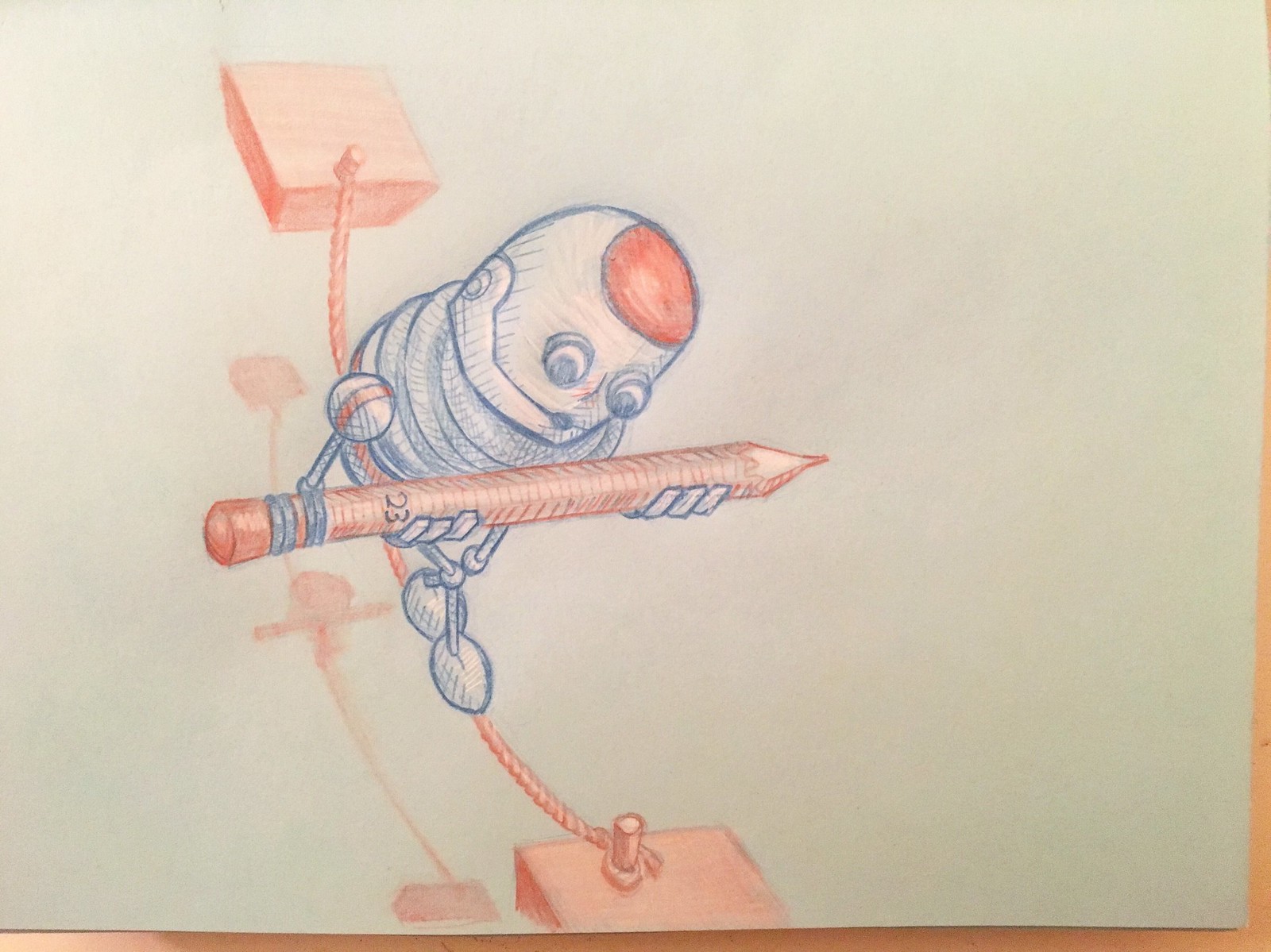This is a highly detailed colored pencil drawing on a piece of white, slightly textured paper, lying against a brown table. It features a skilled and talented depiction of a blue robot walking on a tightrope. The robot has a dome-shaped head with goggly eyes, a red cap marked with the number 23, and a large opening for a mouth that almost looks like a gap. Its body resembles stacked circular rings, giving it a bee-like appearance with its spindly arms and legs ending in small round feet. The robot, carrying a copper-colored pencil inscribed with the number 23, carefully balances on a red line, mimicking a trapeze artist. The tightrope is anchored to two wooden platforms, which appear orange or red, and there are corresponding shadows cast below the robot, the tightrope, and the wooden blocks.